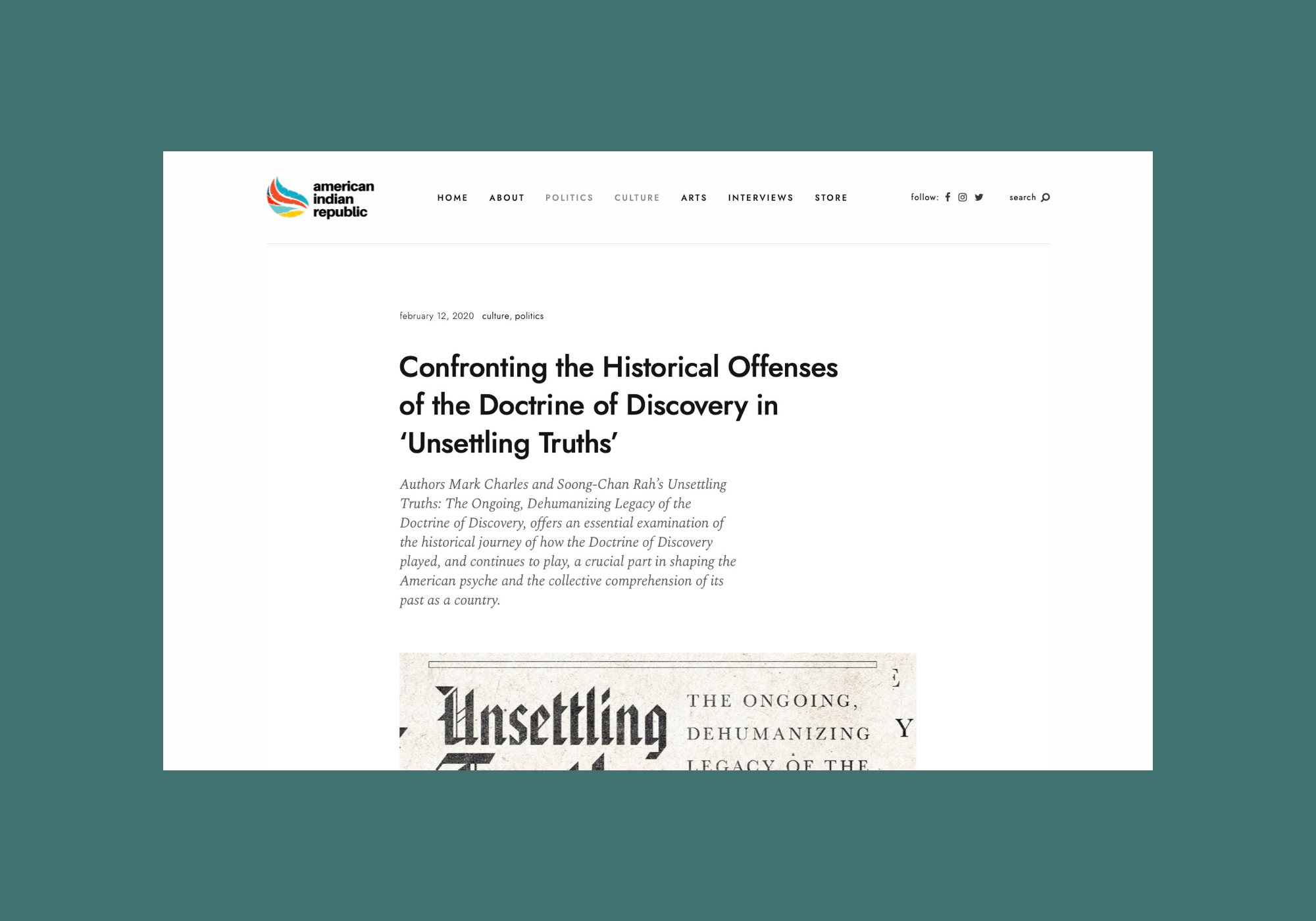The image features a well-designed webpage for the American Indian Republic. Positioned in the upper left corner is a striking stylized logo rendered in shades of orange, red, dark blue, turquoise, light blue, and yellow, resembling feathers. Beside this logo, bold black text spells out "American Indian Republic." 

The top header of the webpage contains black text displaying various navigation tabs labeled: Home, About, Politics, Culture, Arts, Interviews, Store. Notably, the tabs for Politics and Culture are highlighted in light gray, indicating the current sections. Adjacent to these tabs is the label "Follow" in black text, succeeded by dark gray icons for Facebook, Instagram, and Twitter. The header also includes a "Search" label accompanied by a search icon in black text.

Centrally located on the webpage is a blog post-like feature. It starts with a lowercase header that reads "February 12, 2022, Culture / Politics." This is followed by a prominent bold header stating, "Confronting the Historical Offenses of the Doctrine of Discovery in Unsettling Truths." Directly beneath this title, dark gray italicized text provides an insightful summary: "Authors Mark Charles and Sun Ching-Ra's Unsettling Truths, the Ongoing Dehumanizing Legacy of the Doctrine of Discovery, offers an essential examination of the historical journey of how the Doctrine of Discovery played and continues to play a crucial part in the shaping of the American psyche and the collective comprehension of its past as a country."

Below this summary, a grayscale scan of a newspaper is partially visible. The scan features the word "Unsettling" in bold Old English font alongside block letters reading "the Ongoing Dehumanizing Legacy of the."

The background color of the webpage is a deep, rich teal, providing a striking contrast to the text and elements on the page.